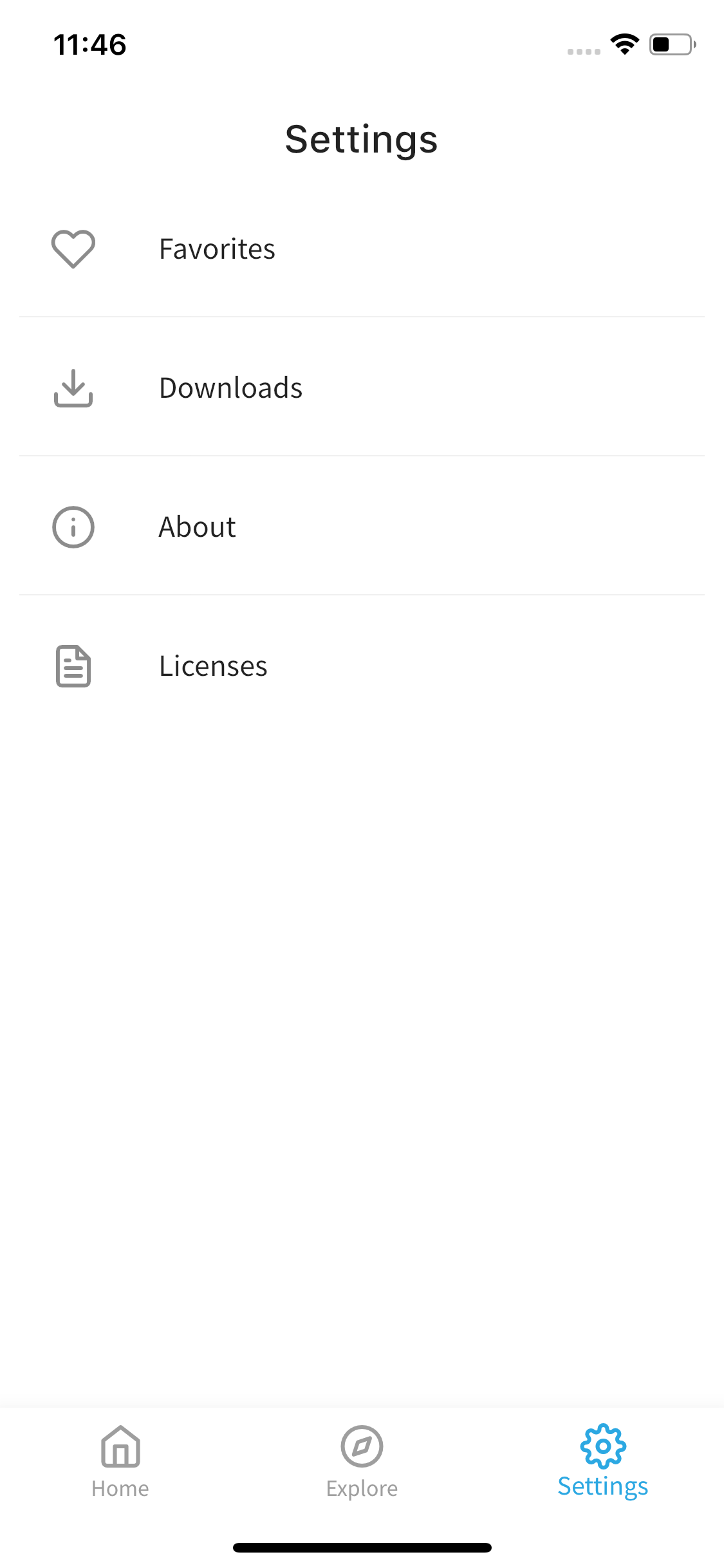In the screenshot, we find ourselves in the settings section of an unidentified app, characterized by its minimalistic and straightforward design. The interface features a clean white background with black text for high readability. At the bottom of the screen are three navigation tabs labeled Home, Explorer, and Settings. The Explorer tab is denoted by an icon that resembles a small compass, hinting it may be related to travel or discovery, although this is not definitively clear.

The settings interface itself provides access to four primary options: Favorites, Downloads, About, and Licenses. Each category allows users to manage respective content, such as unfavoriting items or deleting downloads. This section appears focused on content management rather than altering app behavior or settings.

Additional on-screen elements include a battery icon, showing less than half charge remaining, and a full Wi-Fi signal indicator. The settings tab is represented by a classic gear icon, reinforcing its purpose within the app. This stark, utilitarian design ensures users can quickly navigate and manage their app content with ease.